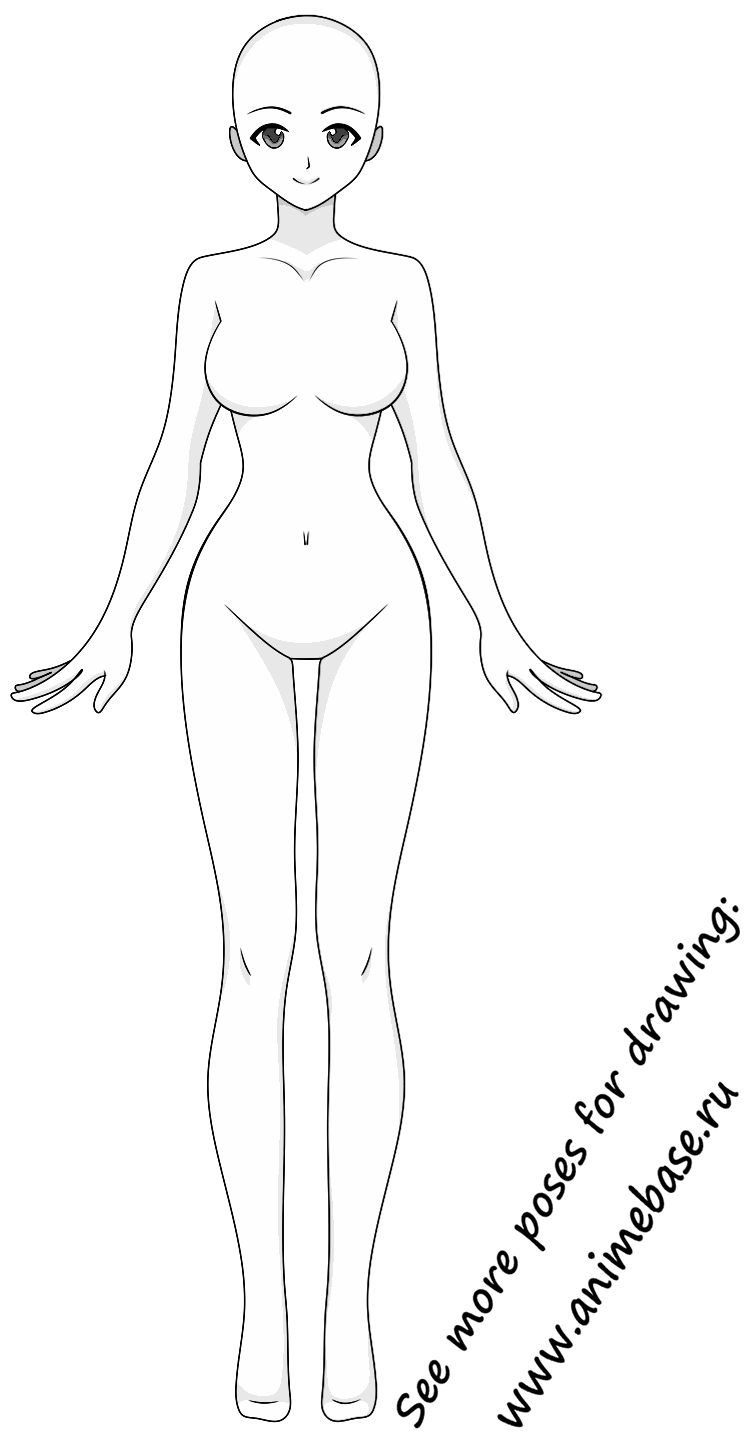This black and white drawing depicts a bald, humanoid female figure standing against a white background, with large eyes, a small nose, and a small mouth. The body has no detailed features, giving it a smooth, mannequin-like appearance, lacking toes and any genital details. The figure has an hourglass shape with pronounced breasts and long legs. Its arms are positioned down by its sides with the fingers splayed outward. There is black text diagonally placed next to her legs on the right side, reading "See more poses for drawing www.animebase.ru."